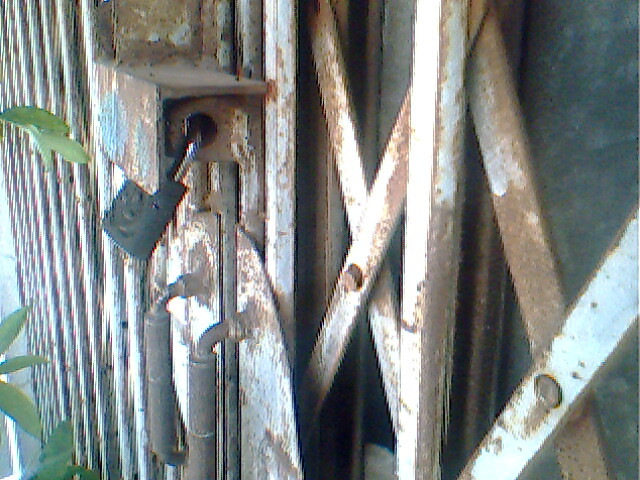The blurred and heavily pixelated outdoor image depicts a rusted metal gate, which is closed and secured with a corroded brown-colored padlock. The light-colored yet rust-stained gate features two black-handled bars, suggesting it opens by sliding. Behind the gate, a dark gray or black wall is visible, partially obscured by the intricate pattern of rusted metal X's. To the left side of the image, green leaves from a small tree or bush emerge, adding a touch of nature to the industrial scene. Additionally, attached to the gate is a structure resembling a birdhouse, adorned with what appears to be a silver and black flag-like object hanging from it. Below this structure, pipes extend into what seems to be a wooden surface situated behind the gate. The image is well-lit, enhancing the contrast between the decaying metal and the natural elements.